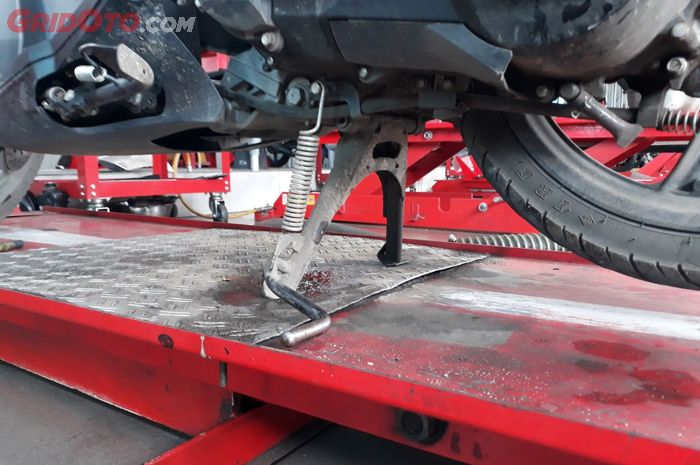A close-up photograph of a motorcycle kickstand reveals intricate details, highlighting signs of wear and use. The kickstand appears aged, coated with dirt and small stones accumulated from extensive riding. A prominent metal spring is positioned on the left side of the kickstand, which features two legs extending downwards. For additional stability, a shiny, backwards L-shaped component extends from the left, laying flat on the ground. The upper portion of the image includes more motorcycle parts, predominantly black in color, with a partial view of the tire. The tire displays partial letters, "I-R-E," suggesting it might spell "tire," although it's partially obscured and upside down. The motorcycle rests on a red ramp, with more red elements visible in the background, creating a striking contrast with the dark components of the motorcycle.